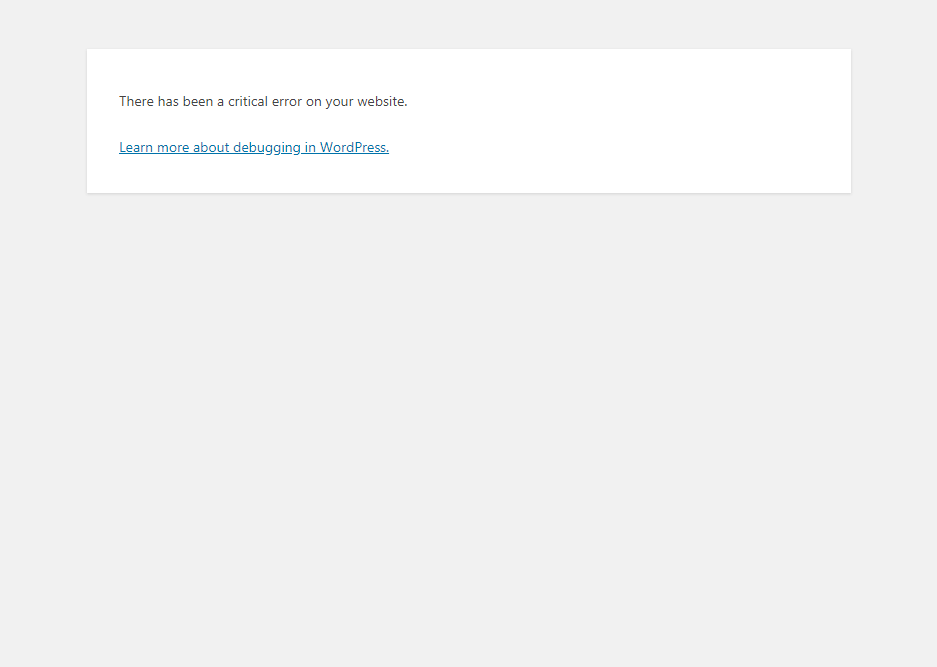The screenshot captures a small section of a webpage displaying a critical error message. The image features a gray background that envelops the entire screenshot. Centrally aligned at the top of the image, there is a neatly spaced, smaller white rectangle containing the core message. The text within the white rectangle is written in black and reads: "There has been a critical error on your website." This message is followed by a line break, creating a clear space between it and the subsequent content. Below the error message, there is a blue, underlined hyperlink that states: "Learn more about debugging in WordPress," which serves as a gateway to further information on troubleshooting the issue. The white rectangle is designed with careful alignment, with both lines of text positioned to the left, contributing to the overall clean and organized appearance of the screenshot.